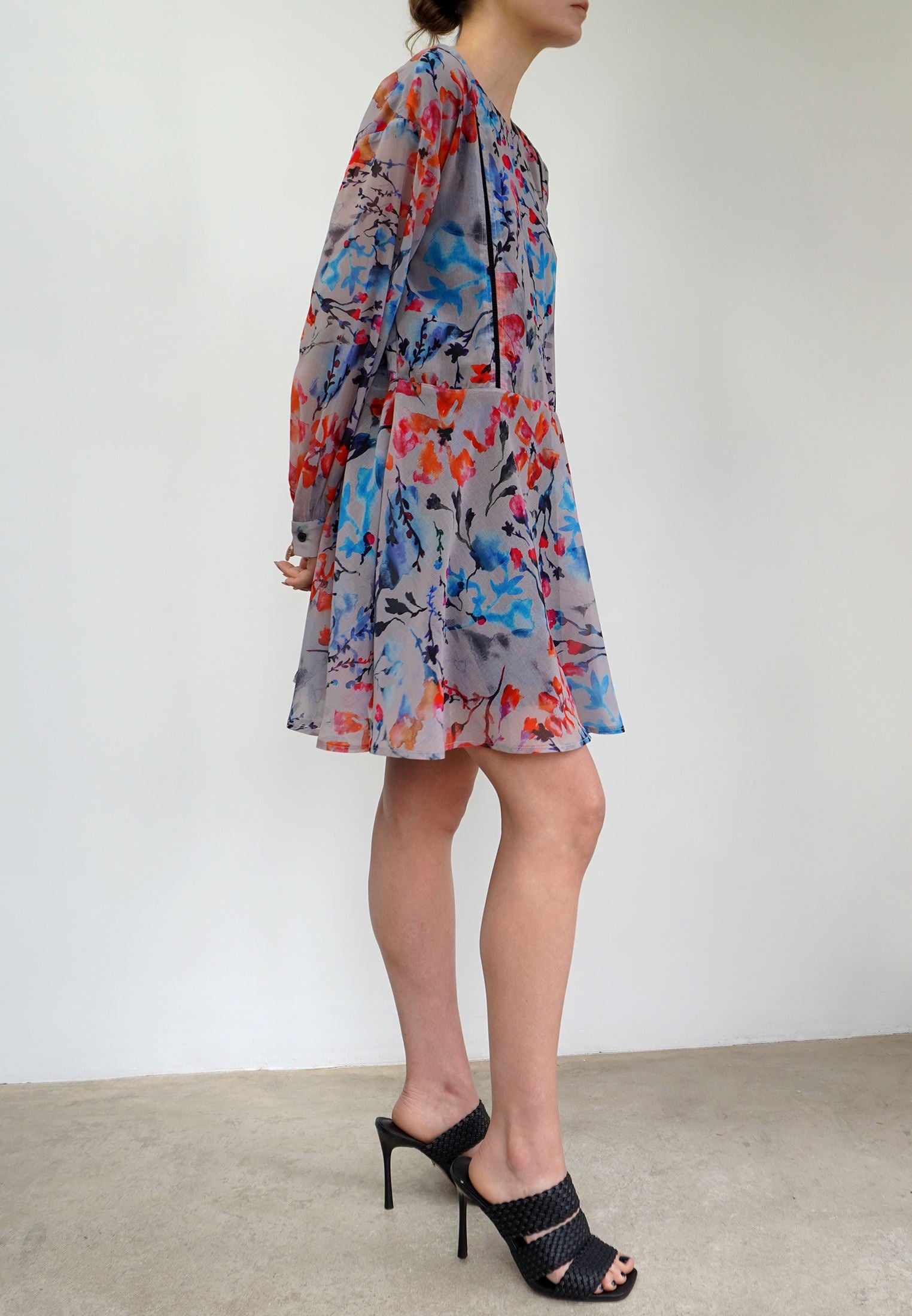This photograph features the side profile of a young Caucasian woman from the chin down to her feet. She stands against a white wall with a beige floor beneath her. She has dark brown hair styled in a bun. The woman is dressed in a gray, flowy mini dress adorned with a pattern of blue, red, and black flowers. The dress, made of light fabric, has long sleeves with button cuffs that appear slightly sheer, revealing a hint of her arm through the material. It cinches at the waist with elastic and extends just above her knees, flaring out with a ruffled hem. Her bare legs lead down to a pair of black leather stiletto sandals featuring three straps across the top of her feet and exposing her toes, which are painted a dark color, possibly navy blue. The image captures her body turned towards the right, showcasing the detailed attire and accessories against the simplistic background.